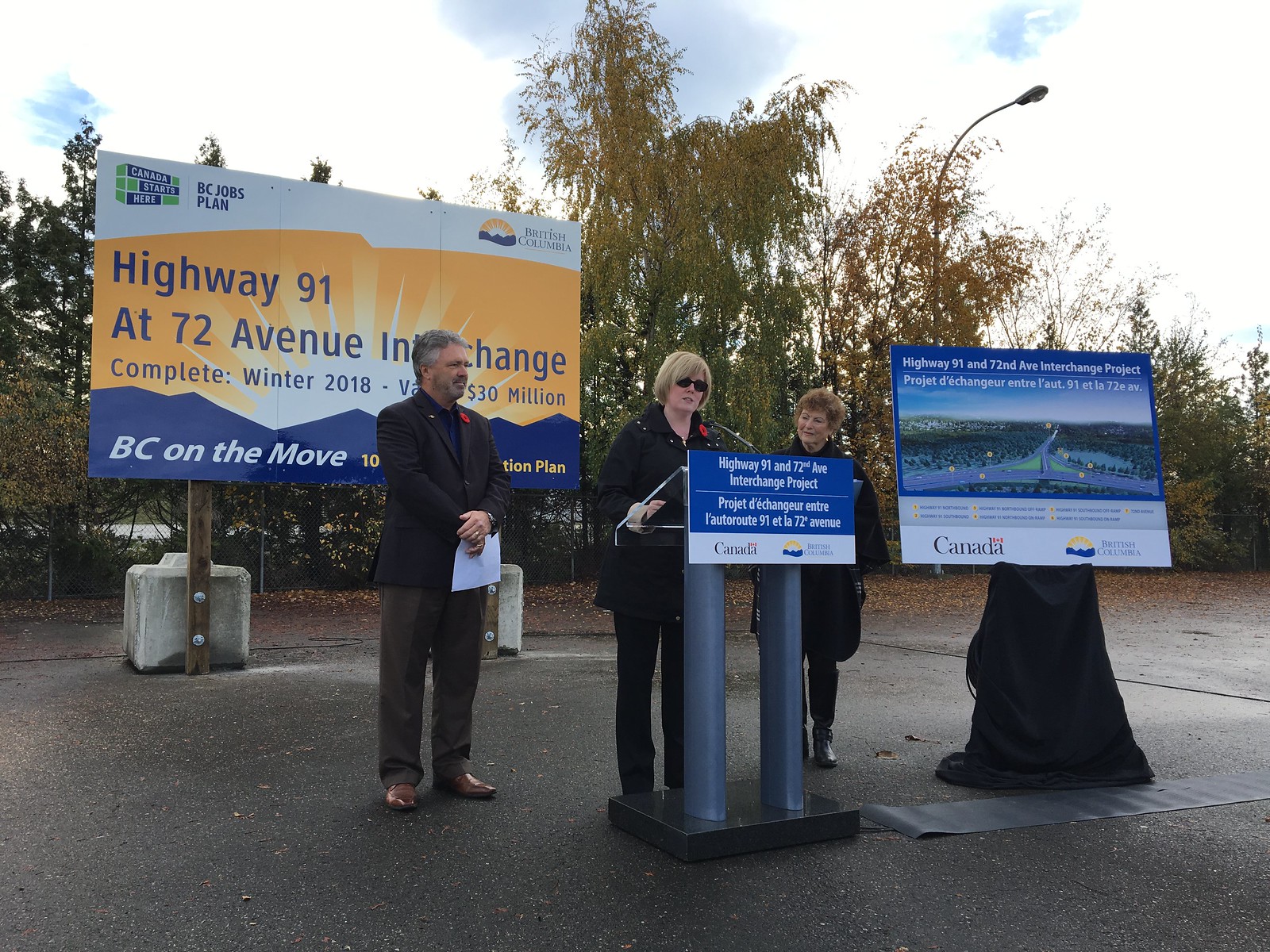A woman with blonde hair, dressed in black, stands at a podium giving a speech. Her arm rests on the podium, which is adorned with a blue sign that reads "Highway 91 at 72 Avenue Interchange Project" and includes a smaller version of the text in either Spanish or French. The sign beneath this states "Canada" accompanied by an image depicting a blue sky, red sun, and some text. To her left stands a man in a black jacket, holding a white piece of paper over his stomach, wearing brown shoes; he likely awaits his turn to speak. To her right is another woman with light brown hair, also dressed in black, with her hands in her pockets. Behind them, a large banner reads "Highway 91 at 72 Avenue Interchange - Complete Winter 2018 - $30 million", and includes the tagline "BC on the move" in gold, white, and blue colors. Another sign to the right features an illustration of the highway project and repeats the interchange project information with additional text about the British Columbia jobs plan.